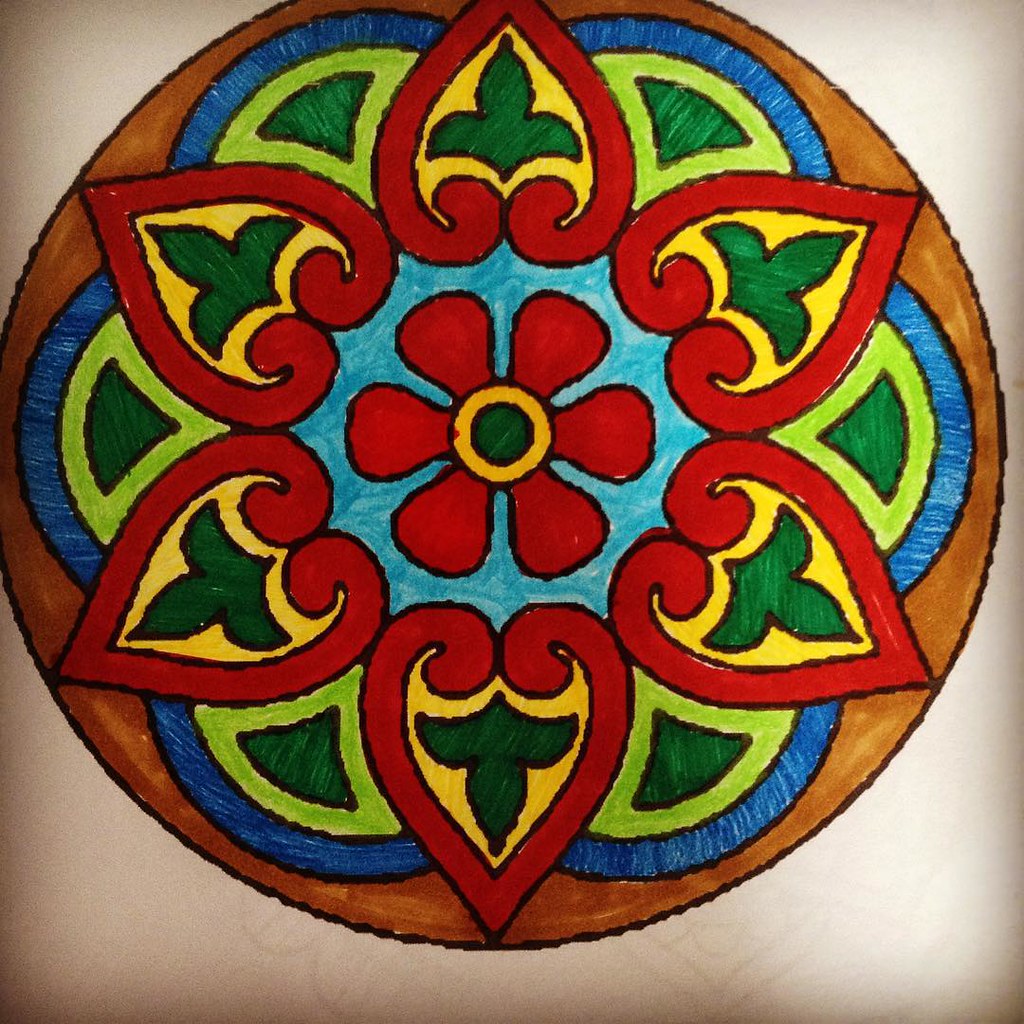This intricate design features a layered, circular composition. At its core lies a solid black circle, encased by a vivid orange ring. Surrounding this is a striking, red six-petaled flower motif. The next layer is a calming light blue ring, which is punctuated with alternating designs of red heart shapes interspersed with yellow segments and green accents. Nestled between the points of the hearts are blue arches complemented by green triangles, adding to the complexity and visual interest of the pattern. The entire design is framed by a beige border, and finally, the outer edge is finished with a rich brown, creating a harmonious yet striking piece of art.